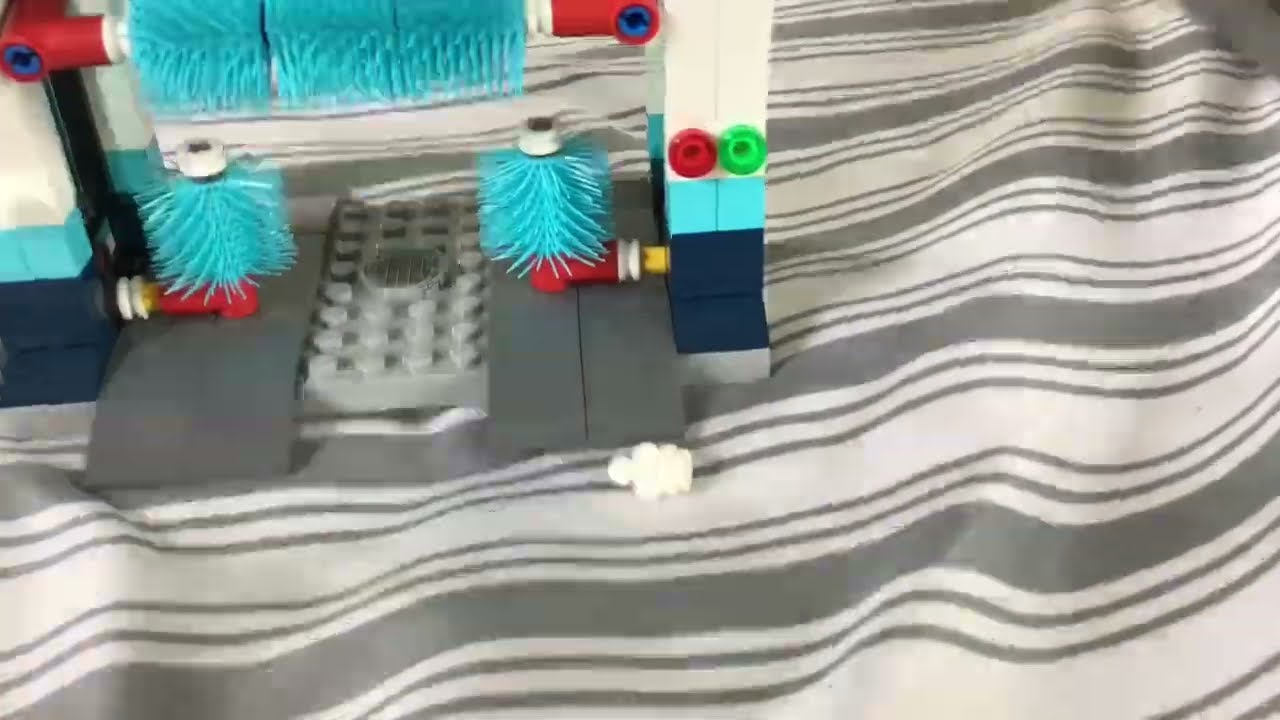This photograph displays a detailed Lego car wash playset positioned on a bed with horizontally striped gray and white sheets. The Lego set features a variety of components, including multiple blue bristled brushes attached in different positions, simulating the cleaning action of a car wash. The structure includes white beams, baby blue, and navy blue blocks, as well as red and green buttons resembling traffic lights. The overall design is complex, with elements such as red arms and turquoise spinning parts, capturing the essence of a miniature car wash. The bed's fabric has a pattern of thick and thin gray and white stripes, adding a textured background to the scene.